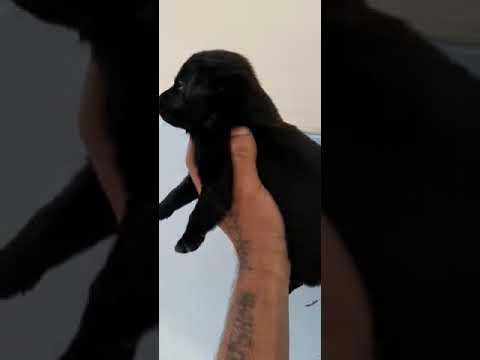In the photograph, a small, black puppy, possibly only a few weeks old, is being held in a man's left hand. The hand, adorned with a black tattoo that spans the top half, cradles the puppy as it gazes to the left. The man's hand is visible from the bottom of the image, but only the lower half of his chin and the upper forearm are seen, without revealing his face or full arm. The background is a white or slightly beige wall, and the image is structured with a central focus where the puppy and hand are prominent, while the left and right edges are darker, zoomed-in sections of the same image, creating a frame-like effect.